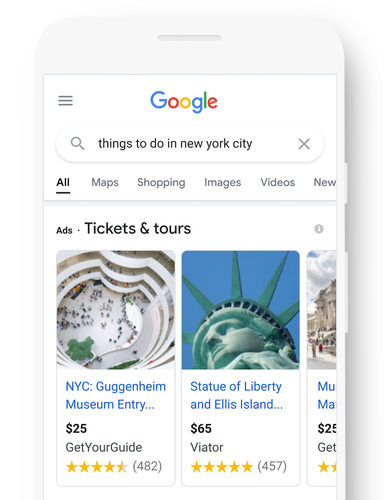A detailed and cleaned-up caption would be:

"This image is a screenshot taken from a white smartphone, which closely resembles an iPhone, capturing about three-quarters of the device. The screen shows a Google search page with the familiar blue, red, yellow, and green Google logo centered at the top. To the left of the logo is the hamburger menu icon. Below the logo, there is a search bar with the text 'things to do in New York City,' flanked by a magnifying glass icon on the left and an 'X' icon on the right. The navigation options below the search bar include 'All,' 'Maps,' 'Shopping,' 'Images,' 'Videos,' and 'News,' with 'All' highlighted and underlined in black.

Further down, there is a section labeled 'Ads' in the top left corner, displaying three images, two of which are fully visible while the third is partially cut off. The first ad is for 'Get Your Guide' and offers tickets and tours starting at $25. The second ad promotes a tour of the Statue of Liberty and Ellis Island for $65, and it includes a five-star rating."